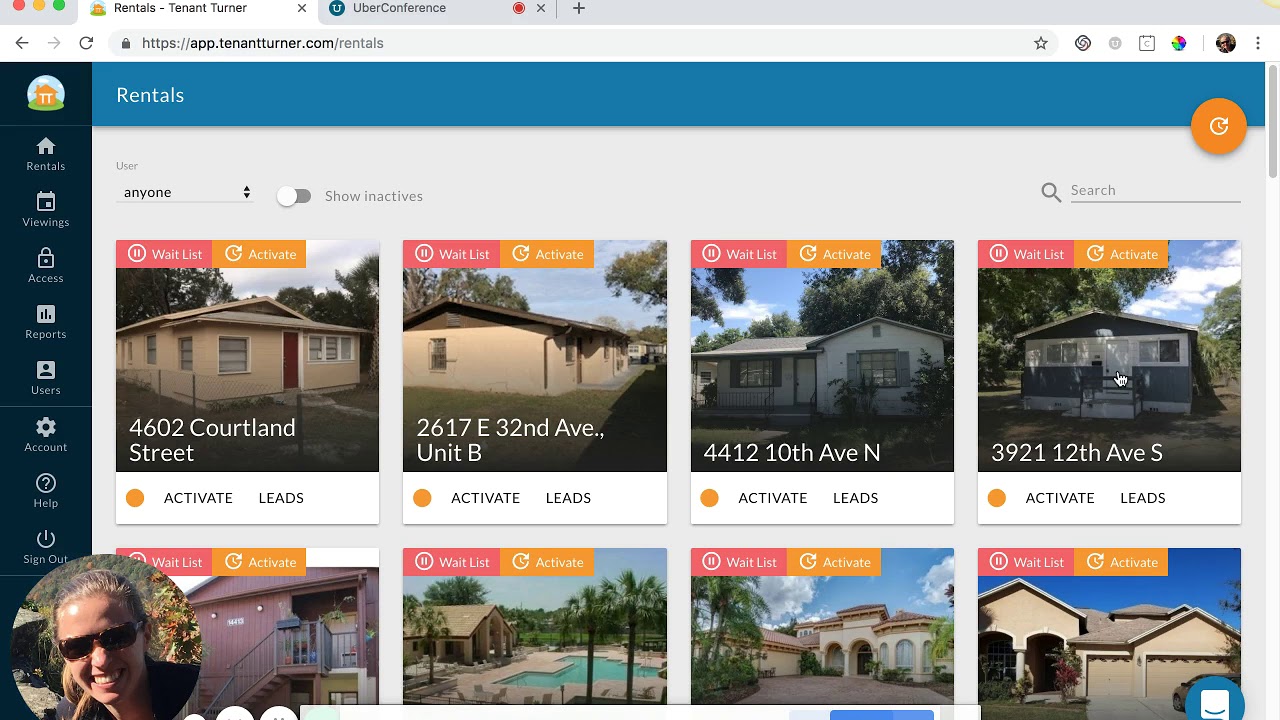A detailed screenshot of a desktop web browser open on a Mac device is prominently displayed. The iconic red, yellow, and green circles in the upper-left corner confirm the operating system. Two tabs are visible: the first labeled 'Reynolds' and the second appears to pertain to a conference. Directly below these tabs sits the web address bar.

The left side of the browser features a vertical black sidebar containing a series of tabs labeled ‘Reynolds,’ along with a comprehensive list of additional options. At the very bottom of this sidebar are buttons for 'Settings' and 'Sign Out.' Positioned in the bottom-left corner of the sidebar is a small photo of a woman smiling broadly, wearing dark sunglasses.

Dominating the main section of the page is a central blue bar labeled 'Rentals.' Below this banner are two rows, each displaying four images, totaling eight property listings. Each property image is accompanied by buttons labeled 'Activate' and 'Leads.' Additional annotations include a small orange button with a timer icon in the upper-right section of the page. Each property image is also tagged with 'Waitlist' and 'Activate' labels in the upper-left corner.